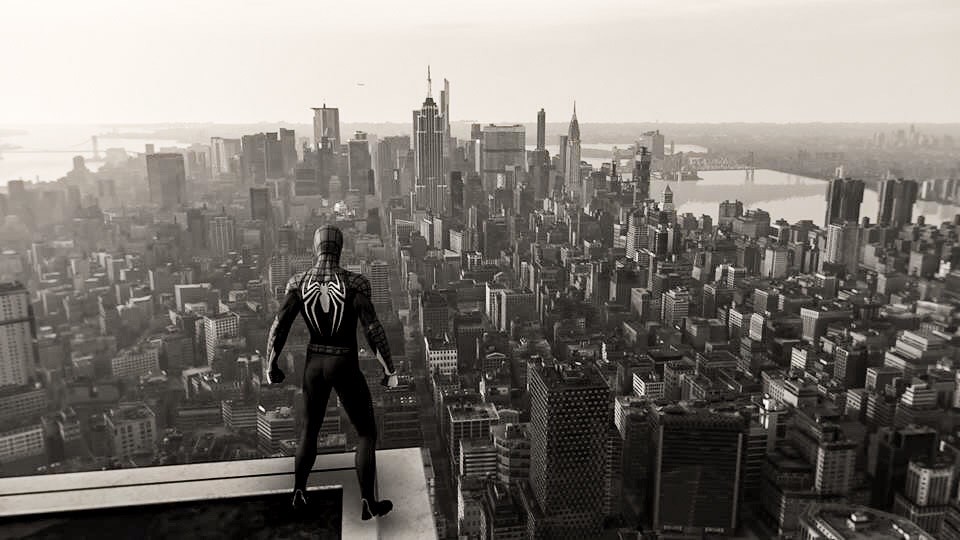This black-and-white image features an intricately detailed 3D model of Spider-Man, likely from Insomniac's game, standing on the edge of a skyscraper's rooftop. Viewed from behind, Spider-Man's distinct spider logo is prominently displayed on his back. He overlooks a sprawling cityscape filled with countless tall buildings and high-rises that stretch endlessly across the horizon. From this elevated vantage point, Spider-Man appears to be contemplating the view. In the background, a large river is visible to the right, and a bridge can be seen on both the left and right sides. The exceptional level of detail in both Spider-Man's model and the cityscape, including individual windows and lights, creates a remarkably realistic scene.